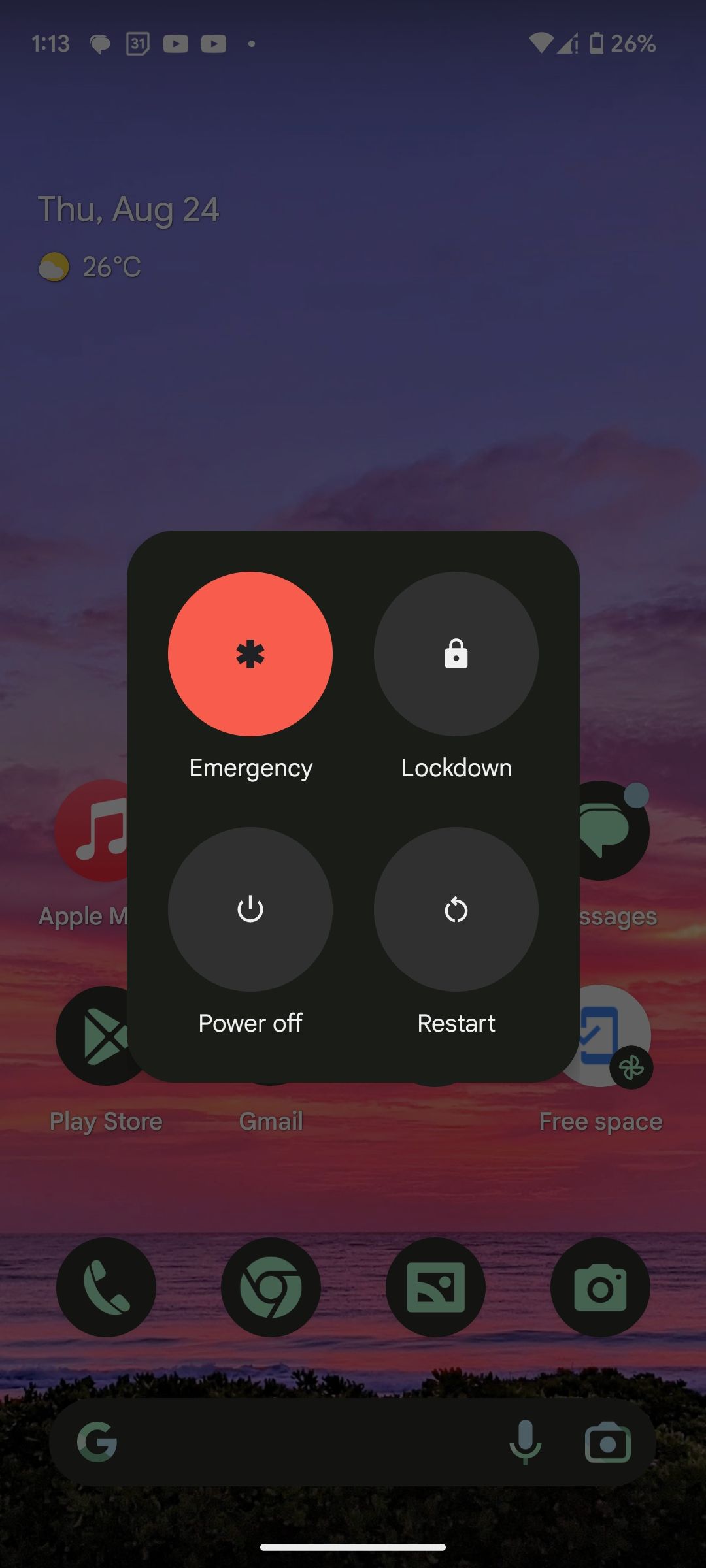A detailed descriptive caption:

In this image, we see a screenshot from a smartphone displaying a pop-up menu located in the center. The pop-up is square-shaped with a black background and consists of four circular buttons arranged in a 2x2 grid. The top left button is red with an asterisk symbol and the word "Emergency" beneath it. The top right button is labeled "Lock Down" and features a lock symbol at its center. On the bottom left, a grey circle shows a power button icon with the words "Power Off" below. The bottom right button, also grey, has the word "Restart" under an arrow forming a circular loop.

In the top-right corner of the image, the battery percentage is displayed at 26%, accompanied by a partially filled battery icon. To its left, the phone's cellular signal strength is indicated, showing one bar short of maximum, while the WiFi signal strength is at full. The time, displayed in the top left corner, is 1:13. Next to it are a message icon and two YouTube icons. Directly beneath this information, the current date reads "Thursday, August 24th," alongside a temperature reading of 26 degrees Celsius.